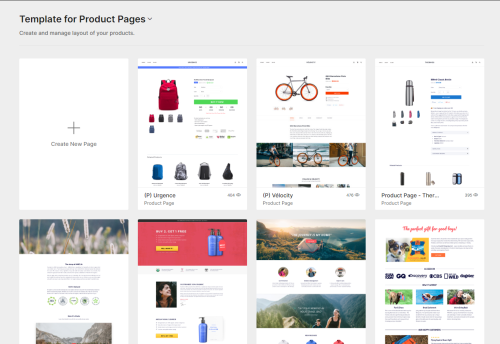In the image, we observe a predominantly gray page, enhanced by several colorful elements. At the top, black text reads "Template for Product Pages," accompanied by a drop-down icon. Below this header, it states "Create and manage layout for your projects."

The first section is a blank page with a white background and a prominent plus sign, labeled "Create New Page." The adjacent page displays a vibrant layout featuring a blue banner, white background, and green buttons. This section showcases various backpacks, including a red sporty backpack with multiple color options such as gray, black, green, and blue. Additionally, there are images of other backpacks in colors like blue, silver, black, and a sling-style backpack.

The following section presents a high-performance sport bicycle designed for distance travel, characterized by orange wheels and a black frame. Beneath this, images depict the bicycle in use, with the text "Velocity" seemingly visible.

The final section displays a silver thermos available in several colors: pink, blue, and silver. Blue buttons at the bottom offer access to different types of thermoses.